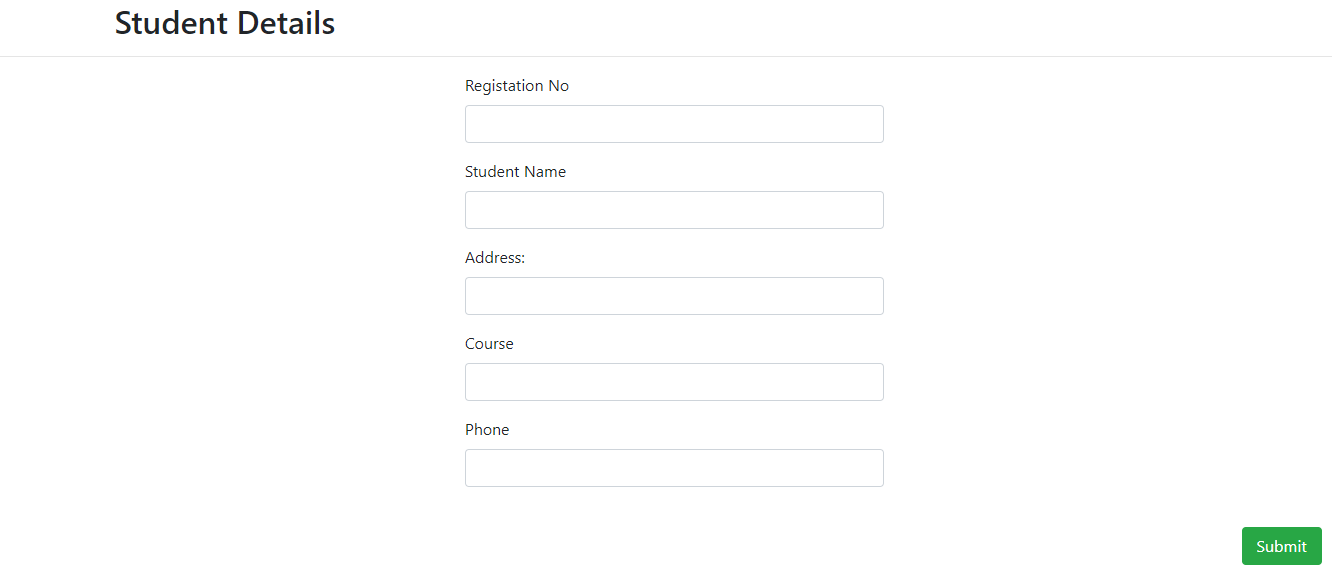The image depicts a remarkably plain and generic student registration form set against a white background. The form's primary header reads "Student Details" in black text, underscored by a gray line. Several black text fields are laid out for user input: the first box, labeled "Registration NO," followed by fields for "Student Name," "Address," "Course," and "Phone." There is no additional context or identifying information such as a school name or logo. The sole distinguishing feature is a green "Submit" button located at the bottom right corner of the page. This undistinguished design suggests the form is meant for basic data collection, possibly to assist in student enrollment or processing.